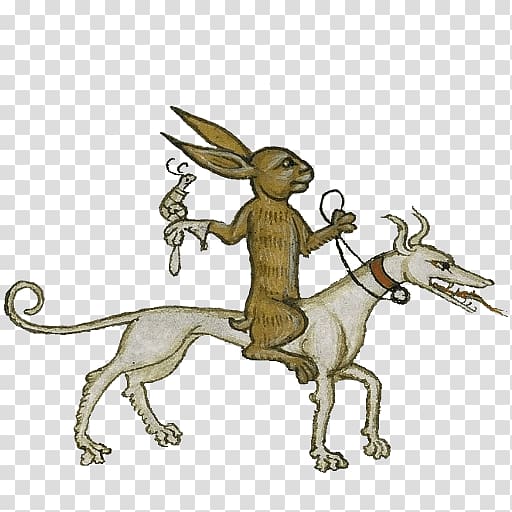The image features a hand-drawn, computer-animated style illustration set against a square, checkerboard background composed of small light gray and white squares. Central to the image is a slender, gray dog with wavy ears that stick up and back, an open mouth with a serpent-like tongue hanging out, and a tail that curls around to its neck. The dog, facing right, wears a brown or red collar with a loop on the front, from which reins extend.

Riding atop the dog is a brown rabbit facing the same direction. The rabbit sits upright, holding the reins in its left hand while its right hand extends backward, sporting a glove on which perches a snail-like creature with curled antennae. The rabbit, dog, and snail are all depicted in a whimsical, cartoonish manner, emphasizing the playful, storybook quality of the scene. The detailed rendering captures the sense of motion as if the rabbit is riding the dog somewhere, adding to the overall charm of the illustration.